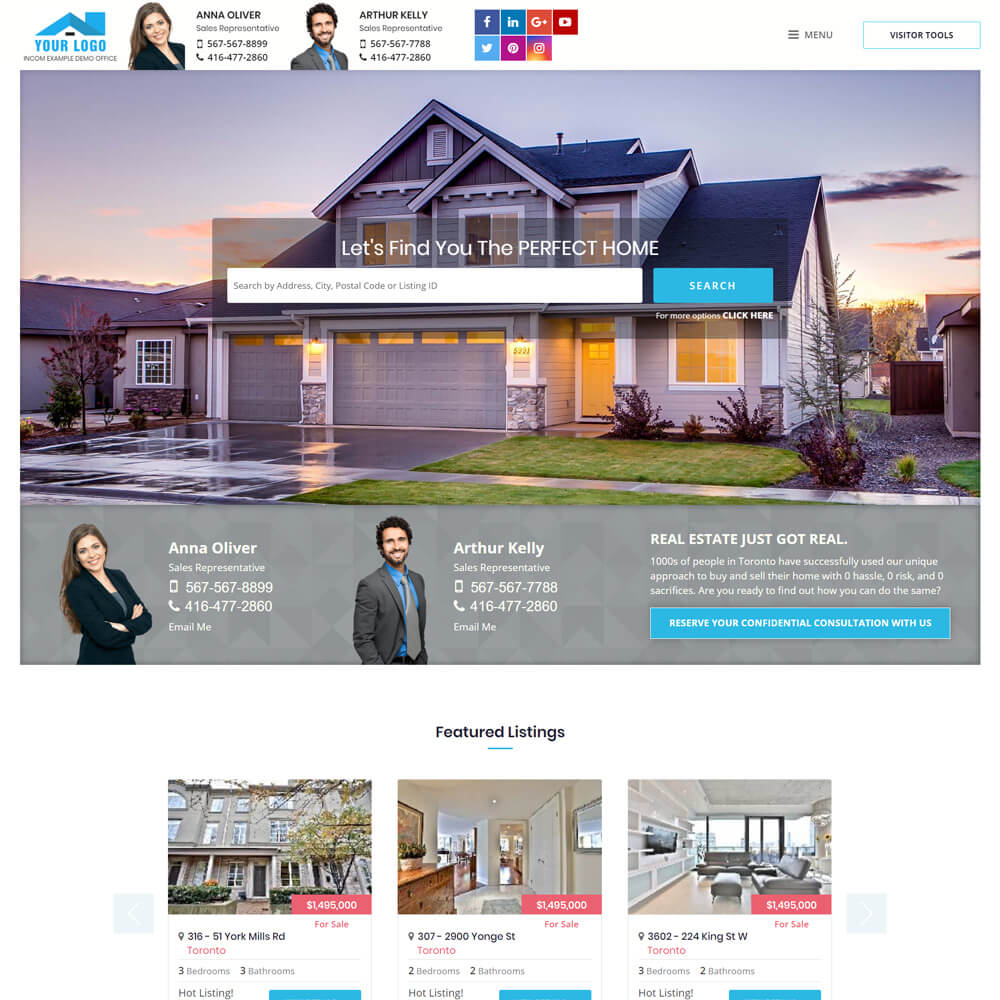The landing page of a real estate website prominently showcases a white background with a central image featuring a picturesque, two-story suburban home at dawn. The house, which boasts a blue thatched roof and beige siding, is illuminated warmly from the inside. The fresh sheen on the driveway, which includes a three-car garage, suggests it either rained recently or the driveway was recently hosed down.

At the top of the page, a banner reads "Your Logo," indicating that this is a mock-up. Beneath, the names "Anna Oliver" and "Arthur Kelly" are displayed alongside their headshots. Both individuals, who have light skin and brown hair, are dressed in business casual attire—Arthur in a gray open-suit jacket with a blue shirt and Anna in a complementary outfit.

The header also includes a navigation menu on the right side, flanked by seven social media icons. The main call-to-action reads "Real Estate Just Got Real," followed by an invitation to "Receive your confidential consultation with us," which is highlighted on a blue button. Below this, the section "Featured Listings" showcases three images of the interiors of different homes, enticing visitors to explore further. The page effectively combines professionalism with a warm, inviting aesthetic.